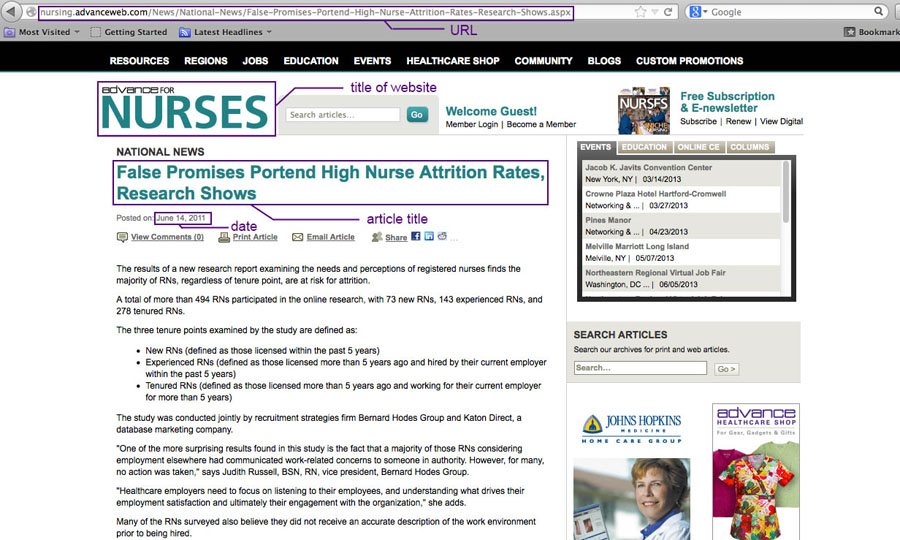**Detailed Caption:**

Screenshot from the website AdvanceWeb.com, specifically its subsection "Advanced for Nurses". The image captures an article titled "National News: False Promises Portend High Nurse Attrition Rates, Research Shows," posted on June 14th, 2011. The screenshot includes various highlighted sections such as the URL, the website title, the article title, and the date of publication for better visual emphasis. The article summarizes the findings of a newly conducted research report on the needs and perceptions of registered nurses (RNs). The research reveals that a substantial number of RNs, regardless of their experience level, are at risk of leaving the profession. The study, conducted jointly by a recruitment strategies firm named Bernard something, indicates that many RNs felt they were not given an accurate portrayal of the work environment before being hired. This points to a concerning trend and the potential future challenges within the nursing profession, driven by unmet expectations and false promises.